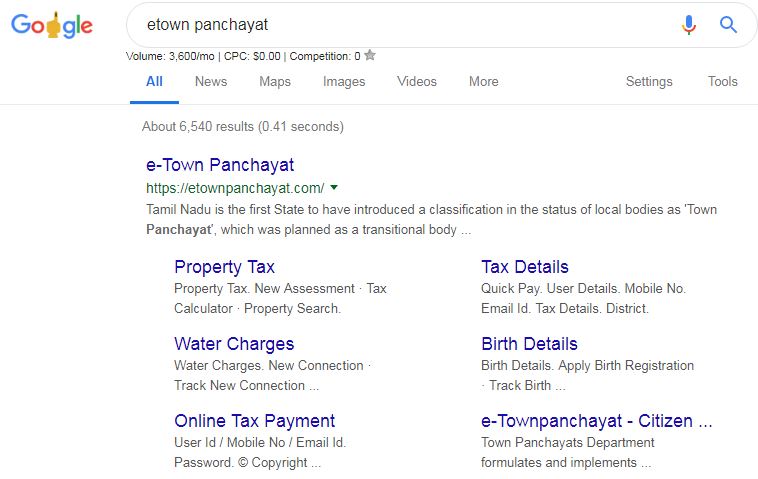This image is a screenshot of a Google search page. The Google logo appears modified, featuring a distinct alteration where the first 'G' in "Google" is replaced by a hand with a finger pointing upward, mimicking the shape of a 'G' but still noticeably different.

The search query entered is "e-town panchayat," displayed prominently in the search bar next to icons for voice search (microphone) and the traditional magnifying glass for text entry. Below the search bar, information on the search volume indicates 3,600 searches per month with a cost-per-click (CPC) value of zero dollars and zero competition, accompanied by a gray star icon.

The navigation links at the top of the page include "All" (currently selected), "News," "Maps," "Images," "Videos," "More," and sections like "Settings" and "Tools." These options provide various filters and tools to refine search results.

The search results area mentions approximately 6,540 results found in 0.41 seconds. The first search result is titled "e-town panchayat" with a URL provided. The brief description states, "Tamil Nadu is the first state to have introduced a classification in the status of local bodies as town panchayat, which was planned as a transitional body..." with an ellipsis suggesting more information is available on the linked page. Below this first result, related topics listed include property tax, water charges, online tax payment, tax details, birth details, and e-town panchayat citizen services.